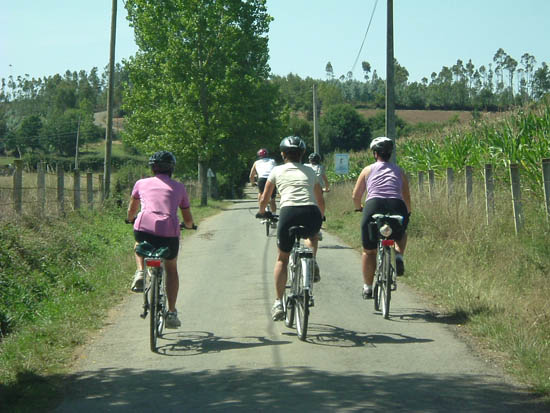The photograph captures five bicyclists riding away on a narrow, barely-paved country road. The road appears grey and dusty, suggesting limited maintenance. Flanked by untrimmed grass, it meanders forward into a slightly hilly area dotted with a mix of trees and open spaces. On either side of the road, wooden or wire fences span between grey poles, possibly securing a crop that looks like corn on the right. Adding to the rural charm, telephone poles with electrical wires stretch along the road. The left side and background are populated by dense trees, contrasted by the light blue sky above. In the foreground, you see three bicyclists closest to the camera and two more further ahead, all riding in the same direction.